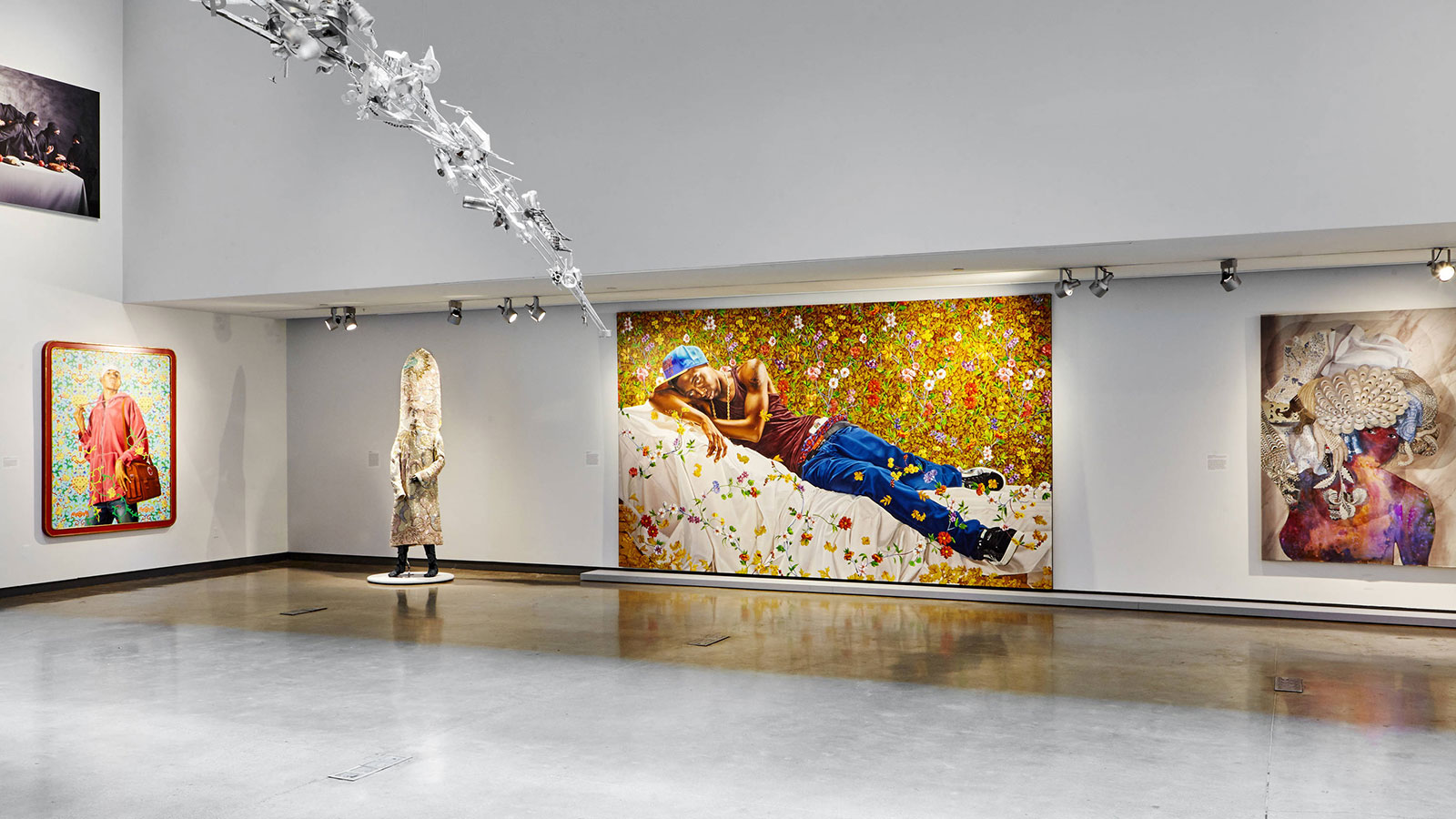The photograph appears to be taken inside a modern art museum featuring white walls with a slight grayish tone, possibly due to the lighting. The floor is made of shiny gray concrete, and there are no people or furniture present. The left wall showcases a painting with a red border, depicting an African American person in a red hoodie and red purse, rendered in a pointillism style. Adjacent to it, there is a large rectangular painting of an African American man lounging on his right side on a bed covered with a white blanket adorned with various flowers. He is wearing a maroon tank top, blue baseball cap, blue jeans, and black sneakers. This painting is illuminated by ceiling lights directly above it. To his left, there is a mannequin-like sculpture dressed in an unusual overcoat with a large head, reminiscent of a finger shape. An abstract painting featuring a large purple mass against white masses is also visible, adding to the museum's eclectic collection.